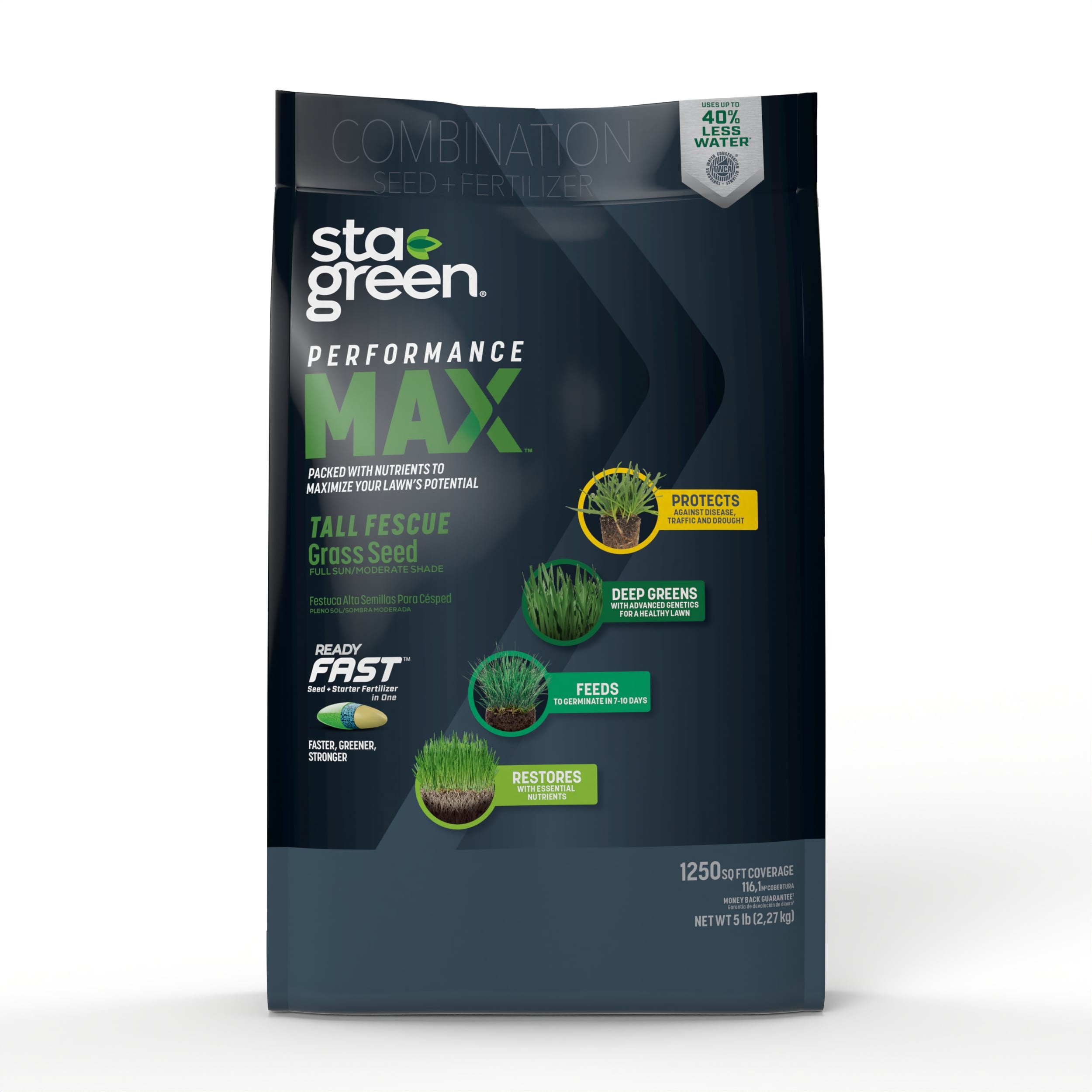This image features a five-pound bag of Stay Green Performance Max grass seed and fertilizer, designed to cover up to 1,250 square feet. The bag, predominantly black and dark gray, is set against a stark white background, highlighting its features. This combination seed and fertilizer is specifically formulated with nutrients to maximize lawn potential, requiring 40% less water. The grass seed is Tall Fescue, known for its fast readiness. The packaging is adorned with four descriptive images each showcasing different benefits: 'Protects' with a yellow circle, 'Deep Greens' with a dark green circle, 'Feeds' with a lighter green circle, and 'Restores' with the lightest green circle. Each image visually represents these benefits with illustrations of thick, healthy grass, ensuring both existing and new grass are lush and resilient.